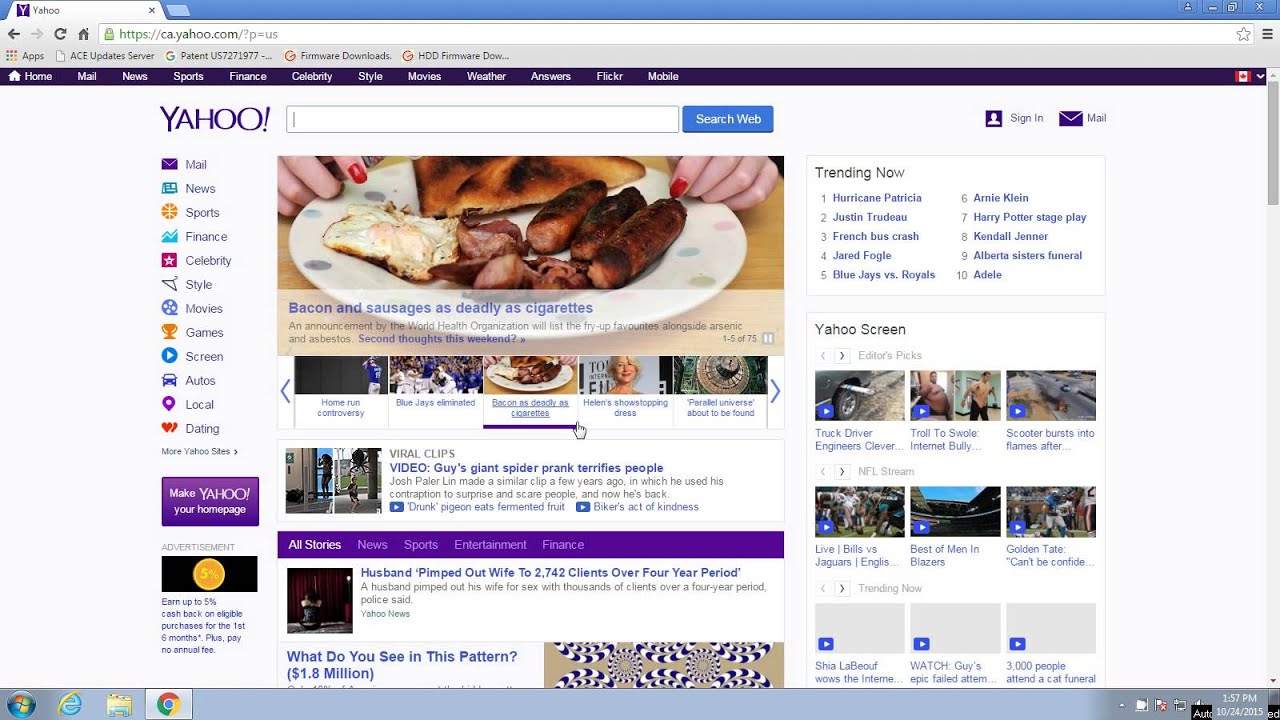This is an image of the Yahoo homepage displayed on a web browser. The browser is set to the Canadian version of Yahoo as indicated by the URL "ca.yahoo.com" and the presence of a Canadian flag on the right, with a downward pointing arrow next to it. The browser has only one tab open, labeled "Yahoo".

The left side of the Yahoo homepage features a vertical toolbar in a purple color with white text. This toolbar includes icons and links for various Yahoo services such as "Home", "Mail", "News", "Sports", "Finance", "Celebrity", "Style", "Movies", "Weather", "Answers", "Flickr", and "Mobile".

To the right of this toolbar, at the top, there is a horizontal navigation bar that includes "Yahoo", a search bar, and options to "Search Web", "Sign In", and "Mail".

Below the horizontal navigation bar, there is another set of categories listed including "Mail", "News", "Sports", "Finance", "Celebrity", "Style", "Movies", "Games", "Streets", "Screens", "Autos", "Local", and "Dating".

The main content of the page features a prominent news article in the center. This article is accompanied by an image of a plate of traditional English breakfast food, which includes items like bacon and sausage. The headline reads, "Bacon and sausage are as deadly as cigarettes," with a subtext mentioning that an announcement by the World Health Organization lists these breakfast favorites alongside arsenic and asbestos.

Additionally, the browser's bookmark bar is visible below the URL, containing items such as "apps", "CE update servers", "patent US 7271977", and "Firmware downloads HDD firmware down". The user appears to be in Canada based on the Canadian flag icon present on the page.